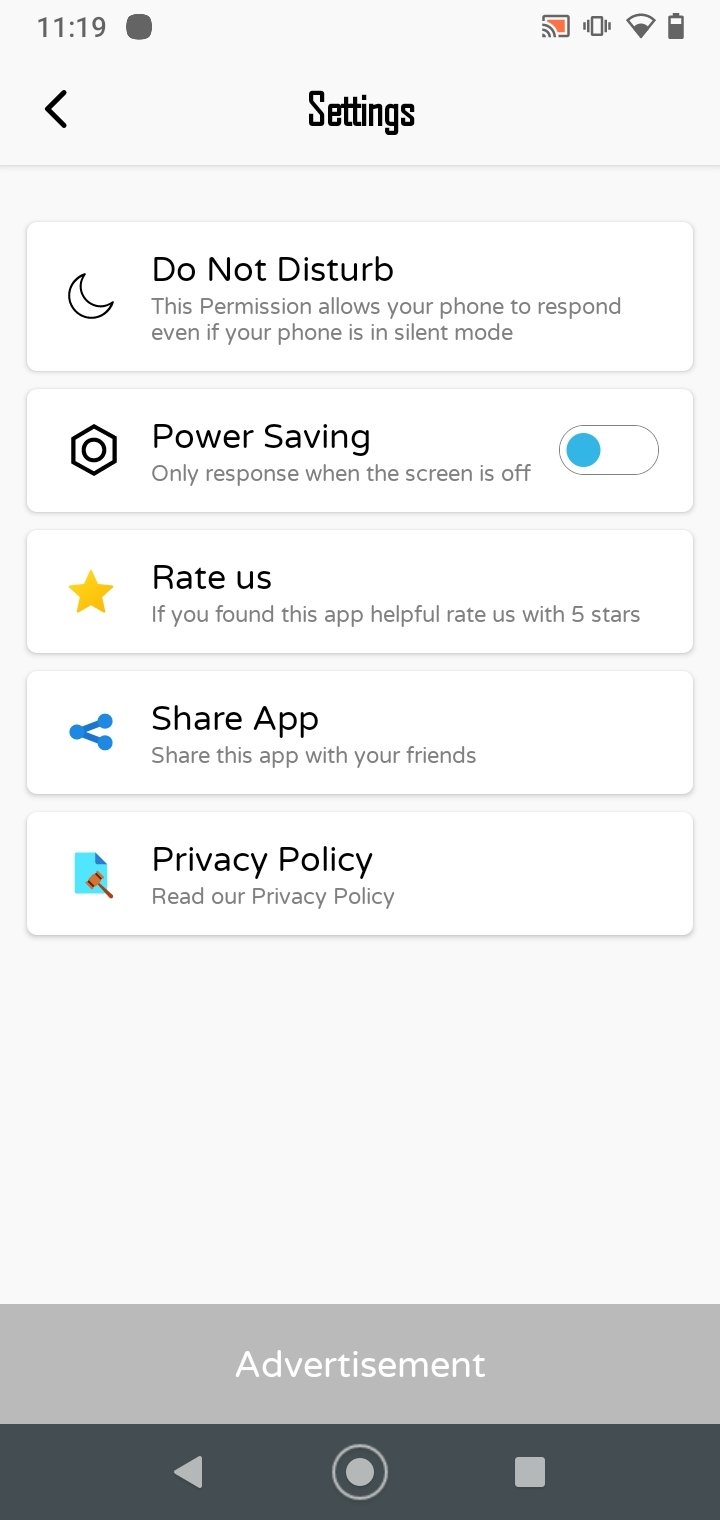The image displays a smartphone screen with a light purple background. At the top of the screen, the time "11:19" is displayed next to a small black dot and a left arrow indicating navigation options. Below this, an icon for settings is present.

A prominent white box contains a "Do Not Disturb" feature, illustrated with a half-moon icon. The caption below the icon explains that this permission allows the phone to respond to notifications even when in silent mode. Additionally, options for power saving and screen-off response are available, and a blue toggle button to activate these settings is visible.

Further down, there is an option to rate the app, symbolized by yellow stars. The text encourages users to rate the app with five stars if they found it helpful. Adjacent to this, a "Share App" option is marked with a sideways V, prompting users to share the app with friends.

The final section contains a blue paper icon and a hammer icon, labeled "Privacy Policy," guiding users to read the app’s privacy policy. The screen's background transitions into a slightly darker purple box labeled "Advertisement."

At the very bottom of the screen, a dark purple navigation bar hosts three icons: a left arrow, a circle, and a square, for additional navigation options.